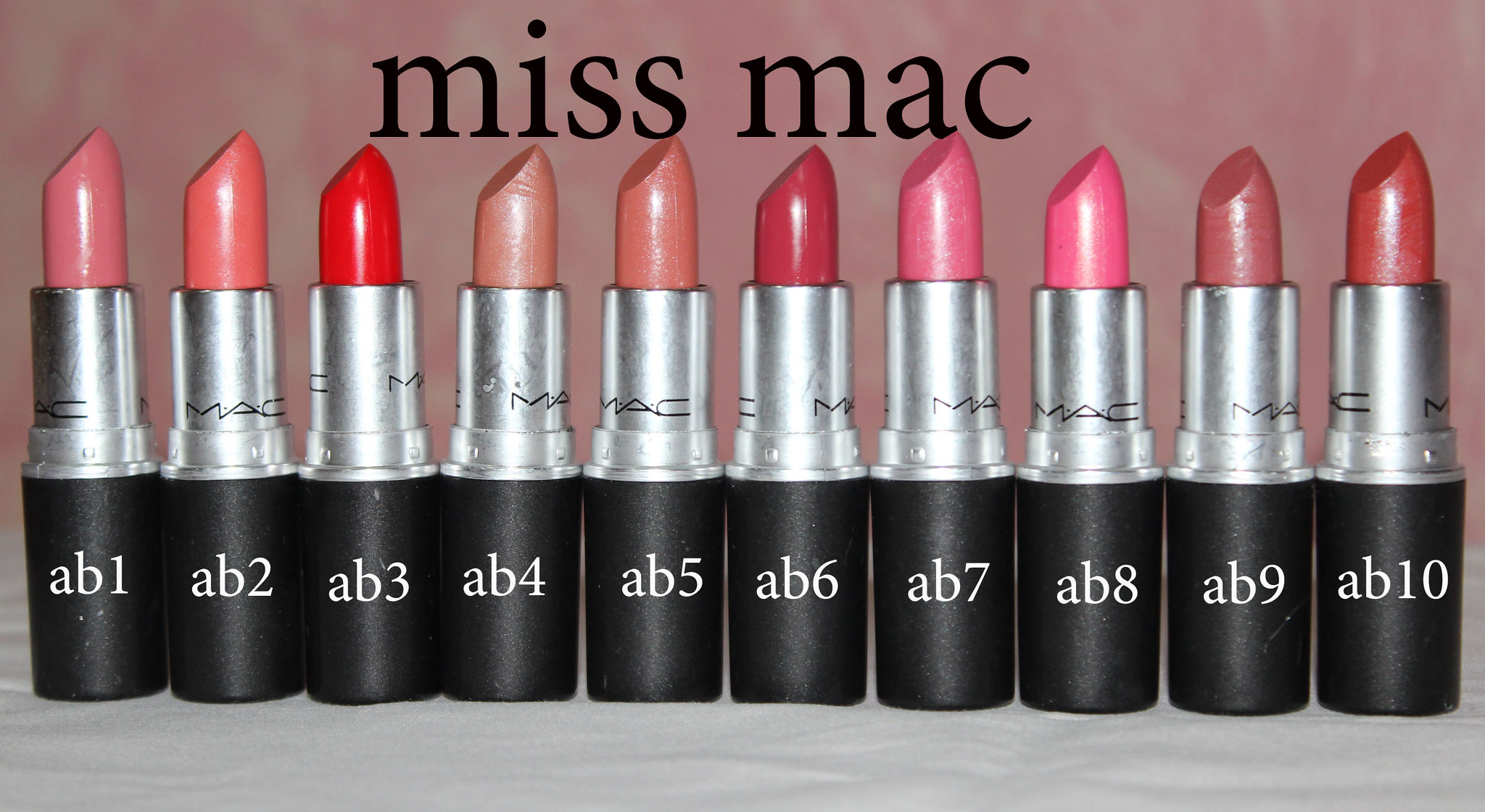This indoor advertisement photograph showcases ten lipsticks from the Miss Mac line, arranged from left to right in neat vertical alignment. At the top of the image, in black lowercase lettering, the brand name "Miss Mac" is prominently displayed. Each lipstick has a sleek black body with a silver, reflective midsection that catches light differently based on their position. On the black section of the lipsticks, there are white labels reading AB1 through AB10. The brand name "MAC" appears in bold, wide black lettering on the silver section. The lipsticks themselves vary in shades, ranging from light pink and tan to various reds and darker pinks, all possessing a cylindrical shape with a flat diagonal top, resembling a crayon. The backdrop of the advertisement features a dark, faded pink hue with hints of gray, adding a sophisticated contrast. The setting is completed with a white cloth at the bottom, which has noticeable folds and creases, adding texture to the overall composition.